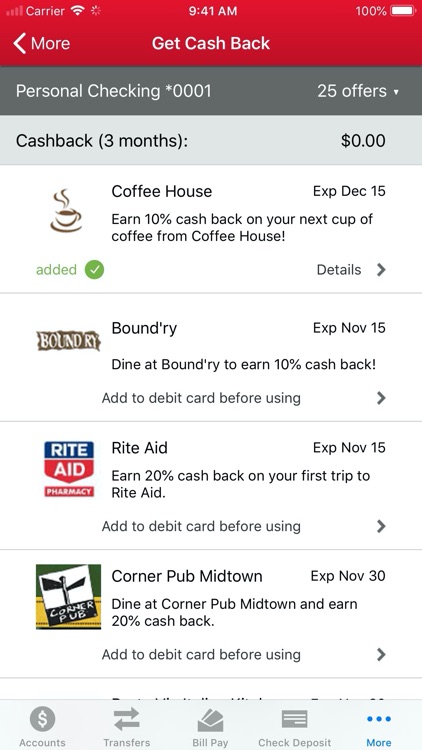The user’s cell phone screen displays a detailed interface with several striking and informative components:

- At the top, a prominent bright red ribbon spans across the screen.
- In the upper left-hand corner, the word "Carrier" appears in white text.
- The center of the screen indicates the time as 9:41 AM.
- To the right, a battery icon shows the battery life at 100%.

Directly below this top section:

- The words "Get Cash Back" are displayed in white text, accompanied by a white back arrow pointing left.
- A dark gray ribbon lies beneath, with "Personal Checking *0001" in white text on the left and "25 offers" followed by a drop-down arrow on the right.

Beneath this dark gray ribbon:

- A light gray ribbon features the text "Cash Back (three months):" with "$0" to the right, both in black text.

Below these headings, the screen lists multiple entries providing cash back offers:

1. A black text entry for "Coffee House" encourages users to "Earn 10% cash back on your next cup of coffee from Coffee House," accompanied by a drawing of a steaming coffee cup to the left. 
   - This offer expires on December 15th.
   - It is marked as "Added" in green text with a green circle containing a white check mark.

The list continues with additional entries such as:

- "Boundary (Stylized as Bound'R-Y)" with its logo to the left.
- "Rite Aid"
- "Corner Pub Midtown"

This detailed user interface is clearly designed to help the user track and maximize their cash back rewards effectively.